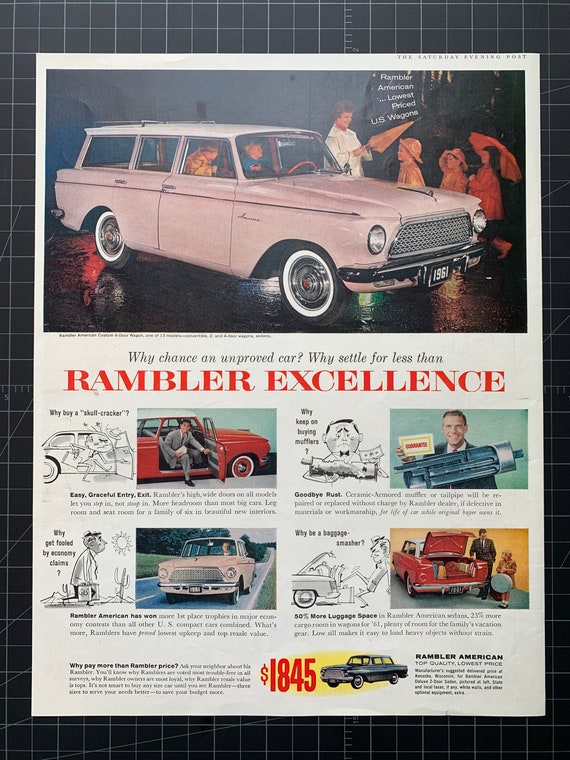This detailed 1960s advertisement for the 1961 Rambler Wagon showcases a vibrant pink station wagon with a white top, prominently displayed at the top third of the page. The vehicle's license plate reads "1961." Inside the car, a man is depicted driving, accompanied by two children in the back seat. Outside, a woman stands holding an umbrella, indicating an interaction amid classic family imagery. As we move down the page, the slogan "Why chance on an unproved car? Why settle for less than Rambler Excellence" is highlighted, with "Rambler Excellence" prominently displayed in large red type.

The ad also includes a secondary image of a man getting out of a red car, juxtaposed with a cartoon illustration of someone struggling to exit a different vehicle. To the right of this, a man holds a steel tube. Below these images, additional views of the Rambler are shown: a pink car demonstrating its impressively spacious trunk and another red car driving, presumably illustrating its smooth performance.

Set against a white page with a black border, the advertisement concludes with the price of $1,845 marked in red text on a yellow background, emphasizing the affordability of the Rambler American. The overall layout and vivid details are designed to capture the viewer's attention, highlighting the superior features and family-friendly aspects of the Rambler Wagon.